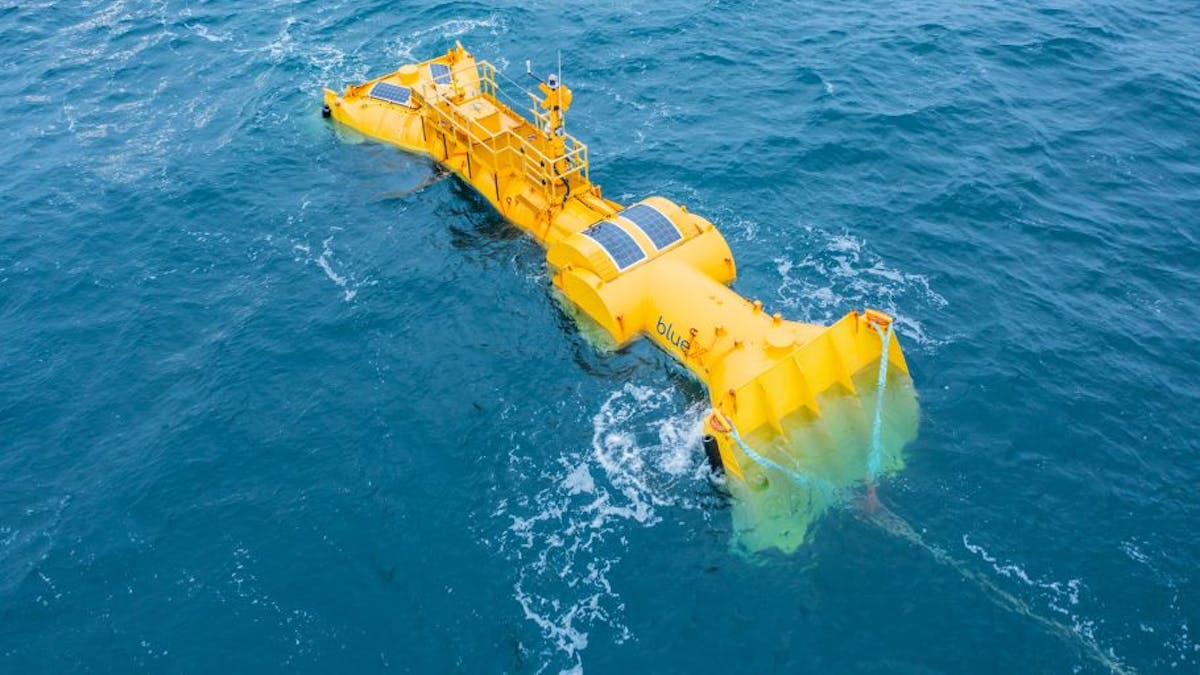The image depicts a long, narrow piece of yellow construction equipment partially submerged in teal blue-tinted water, with no land in sight. The machinery, viewed from above, features a shovel-like appendage at its front-right end, angled flat surfaces with partitions, and a circular extension in the middle. The middle section also includes solar panels situated on a rounded dome, and in between these panels, there's a caged area where a person in a yellow jumpsuit and helmet is visible. The equipment has the word "blue" written in blue ink just behind its forward section on the left side. Surrounding the machinery, the water shows signs of disturbance, indicative of its presence and activity. At the rear, a section of railings suggests a workspace, possibly for a mechanic or operator, and a radar antenna extends upward. This setup could be part of a sophisticated marine research or construction operation, using scientific tools to interact with the underwater environment.